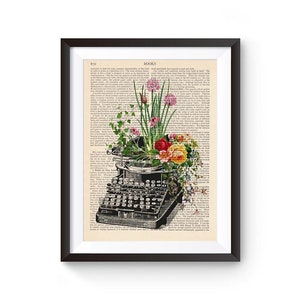This framed image features a striking composition of a black-and-white old-fashioned typewriter and a vibrant bouquet of fresh, spring-colored flowers. Centered on a page of small, indistinct newsprint text, the typewriter appears slightly worn with some broken gray keys. From the top of the typewriter, a diverse floral arrangement of mostly roses with lush greenery and additional flowers in hues of purple, yellow, red, blue, and pink, elegantly drapes downward. This intricate setup is encased within a refined, thin black frame accompanied by a white matting inside, adding an extra touch of elegance to the display.